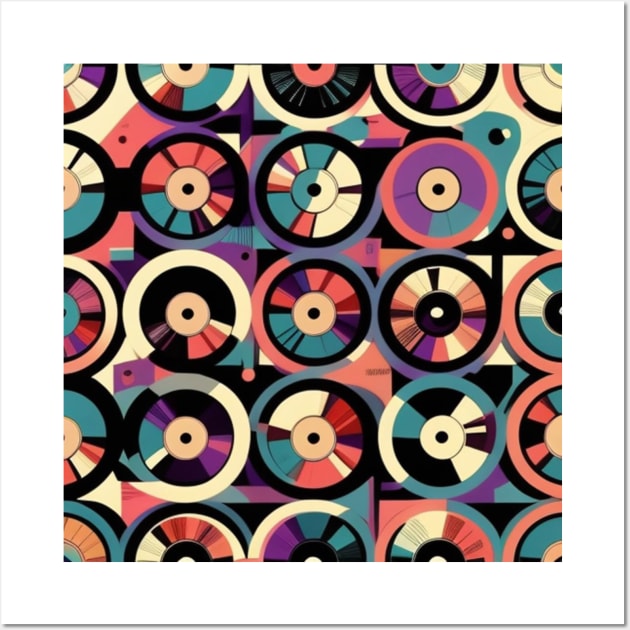This vibrant image evokes a 60s flashback with its striking depiction of LP-like records arranged in a grid pattern. The artwork features five rows and five columns of round discs, with the records along the edges partially cut off. Each disc showcases a variety of muted colors including blacks with brown labels, bands of rainbow-like hues, aquas, blues, purples, reds, oranges, greens, and grays. The records have concentric circles in the middle, giving them a wheel-like appearance. The entire composition is set against a backdrop of abstract, mosaic-like patterns in an array of colors, creating an abstract and colorful effect without any solid backgrounds. A clean white border frames the image, further emphasizing its elegant simplicity and lack of text or writing.